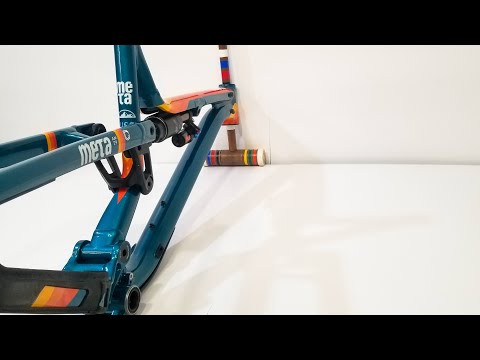The photograph captures an enigmatic metallic structure, primarily colored in aqua or dark teal, positioned against a pristine white floor and wall backdrop. The image is bordered in black at the top and bottom. Central to the composition is a multi-colored mallet, displaying stripes of brown, yellow, green, red, and white, reminiscent of either a polo mallet, cricket bat, or croquet mallet. The mallet leans against the wall, its head resting on the floor. Attached to or converging with the mallet is the metallic structure, which includes several tubular bars. These bars, adorned with stripes of pink, yellow, orange, red, and blue, add to the intricate and colorful design. The word "meta" is inscribed on the tubing, though its exact function remains unspecified. The sterile white setting accentuates the vibrant colors and complex arrangement of the elements within the photograph, creating a visually striking and thought-provoking image.